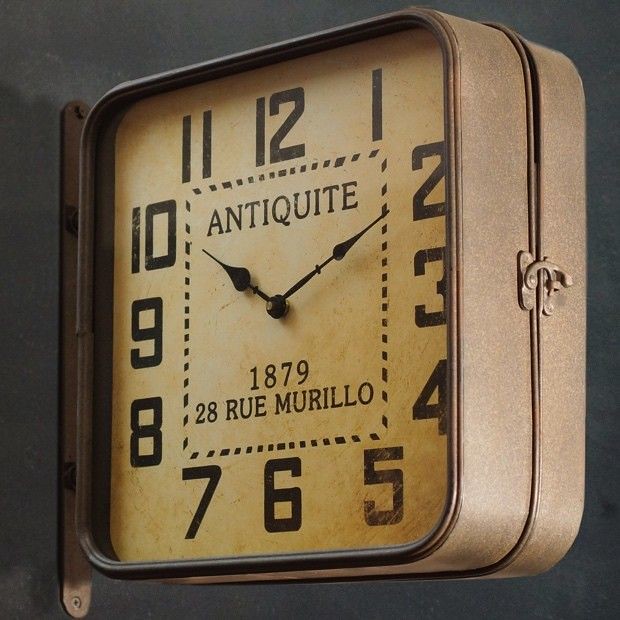This is a detailed square color photograph of a distinctive clock mounted on a grey wall. The clock, which appears to be a modern reproduction of an antique design, features straightforward black Arabic numerals on a yellow background. The clock has a squarish form with rounded edges and is surrounded by a bronzish brown metal casing. Notably, the clock is attached to the wall via a vertical metal bracket of the same brown color, secured with screws.  

Within the clock's face, the word "Antiquité" is prominently displayed repeatedly at the center, while the text "1879, 28, Rue Morillo" is inscribed below, both in black ink. The time shown is 10 past 10, with old-fashioned, black clock hands that are pointy at the front and rounded at the base, anchored by a screw designed to look antique. 

On the right-hand side of the clock, there's a hook or lock mechanism, suggesting that the clock can be opened, allowing access to set the time. Overall, the clock's design exudes an ancient vibe, merging aesthetic charm with historical elegance.